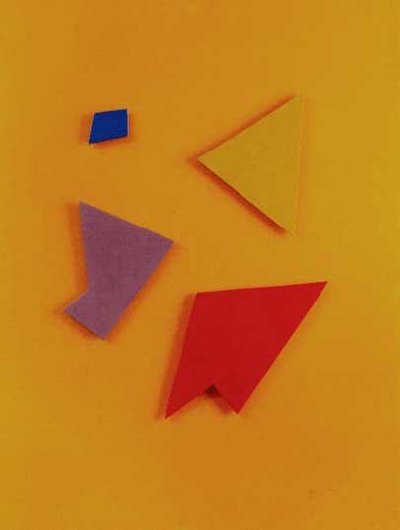The image is an abstract and geometric painting with a vibrant and saturated color palette. It has a portrait-oriented rectangle background in a bright to burnt orange hue. Centered on this background are four distinct geometric shapes:

1. **Top Left:** A nearly square, small trapezoid shape in bright royal blue.
2. **Top Right:** A large, light yellow-orange triangle with a striking red border.
3. **Bottom Right:** A bold, bright red five-sided shape.
4. **Bottom Left:** A purple five-sided figure, formed by two triangles meeting in the center.

Each shape casts a visible shadow, creating a sense of depth against the bright background. The spatial arrangement and colors emphasize the geometric abstraction of the composition.